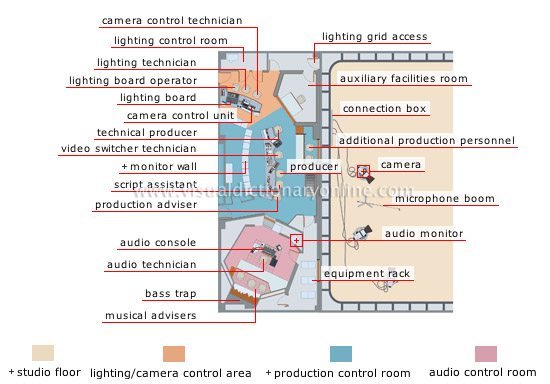This image is a detailed, color-coded floor plan of a TV talk show's recording studio, featuring various technical and production areas. The layout includes multiple locations and equipment placements with color codes at the bottom for reference: tan for the studio floor, gold for the lighting/camera control area, blue for the production control room, and pink for the audio control room.

On the left side of the diagram, labeled items include the Camera Control Technician, Lighting Control Room, Lighting Technician, Lighting Board Operator, Lighting Board, Camera Control Unit, Technical Producer, Video Switcher Technician, Monitor Wall, Script Assistant, Production Advisor, Audio Console, Audio Technician, Bass Trap, and Musical Advisor. On the right side, the labeled items are Lighting Grid Access, Auxiliary Facilities Room, Connection Box, Additional Production Personnel, Producer, with the Camera positioned behind the producer, Microphone Boom, Audio Monitor, and Equipment Rack.

The objects are labeled with words and lines pointing to their positions on the diagram, making it easily navigable for understanding the placements and roles within the studio.